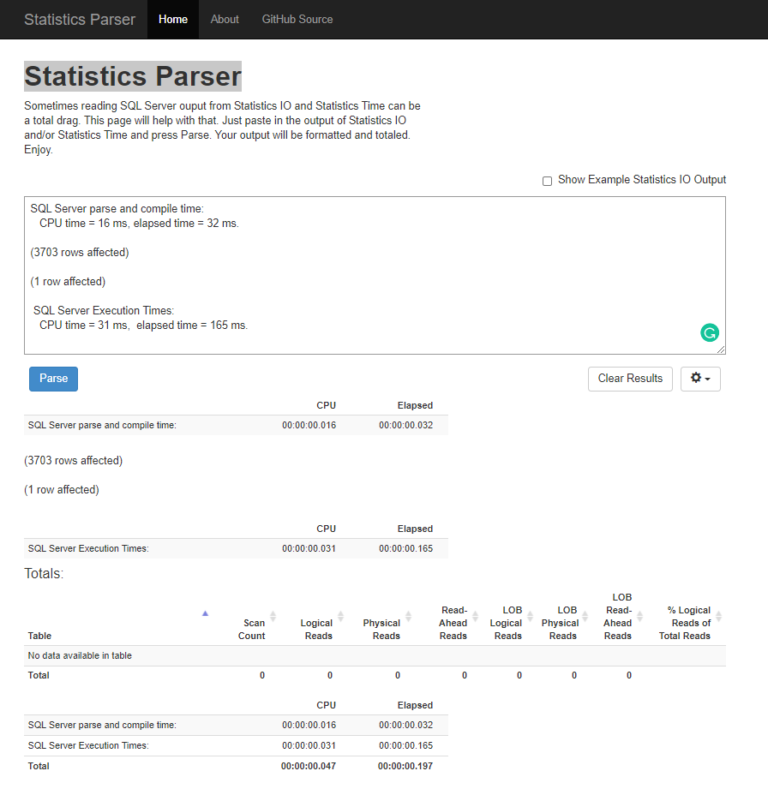The image features a user interface for a tool named "Statistics Parser." The top section of the interface has a black background with various buttons and labels in different colors. At the very top, grey text reads "Statistics Parser." This is followed by a white "Home" button, then more grey text reading "About" and "GitHub Source."

The main content area of the interface has a white background, with a grey section featuring black text that introduces the tool as "Statistics Parser." The text explains the tool’s purpose: solving the tedious task of reading SQL Server output from "Statistics I.O." and "Statistics Time." The instructions specify that users can paste output into the designated area and press "Parse" to have the output formatted and summarized. 

To the right side, there is an example output box showing sample SQL Server statistics, including metrics like CPU time and elapsed time in milliseconds, and rows affected. Specific sample data includes "SQL Server Time, CPU: 16 milliseconds, Elapsed Time: 32 milliseconds, 307 rows affected" and another entry showing "SQL Server Time, CPU: 31 milliseconds, Elapsed Time: 165 milliseconds."

Below the example box, there are buttons for additional functionalities such as a "Pause" button, a "Clear Results" button, and a "Functions" feature. The diverse layout is further complemented by various sections containing a mix of grey and white backgrounds, with black text that delves into more technical specifics related to computer and SQL operations. The caption concludes with the user admitting difficulty understanding some of the technical details described in the black text on the different colored backgrounds.